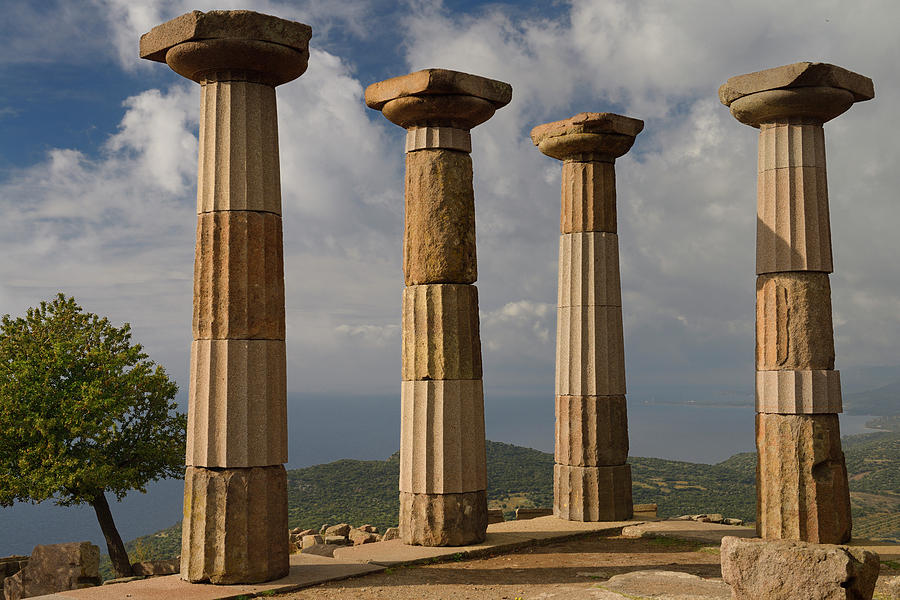The image depicts ancient ruins situated on a hilltop, featuring four towering stone columns. Each column is segmented into four or five sections, with some displaying a striped pattern of alternating colors, while others remain plain. These monumental columns are topped with flat, square stone pieces, creating a striking silhouette against the sky. The scene overlooks a lush valley with verdant hills and dense vegetation, including a prominent leaning tree on the left side, possibly an olive tree. In the distant background, the ocean stretches out under a canopy of clouds, adding to the timeless feel of the landscape. The ruins, likely from an ancient European civilization, exude an air of antiquity and dominance, reminiscent of ancient Roman sites such as those found on Crete. Surrounding the columns are various scattered stones and bricks, set upon an extensive, flattened stone platform.